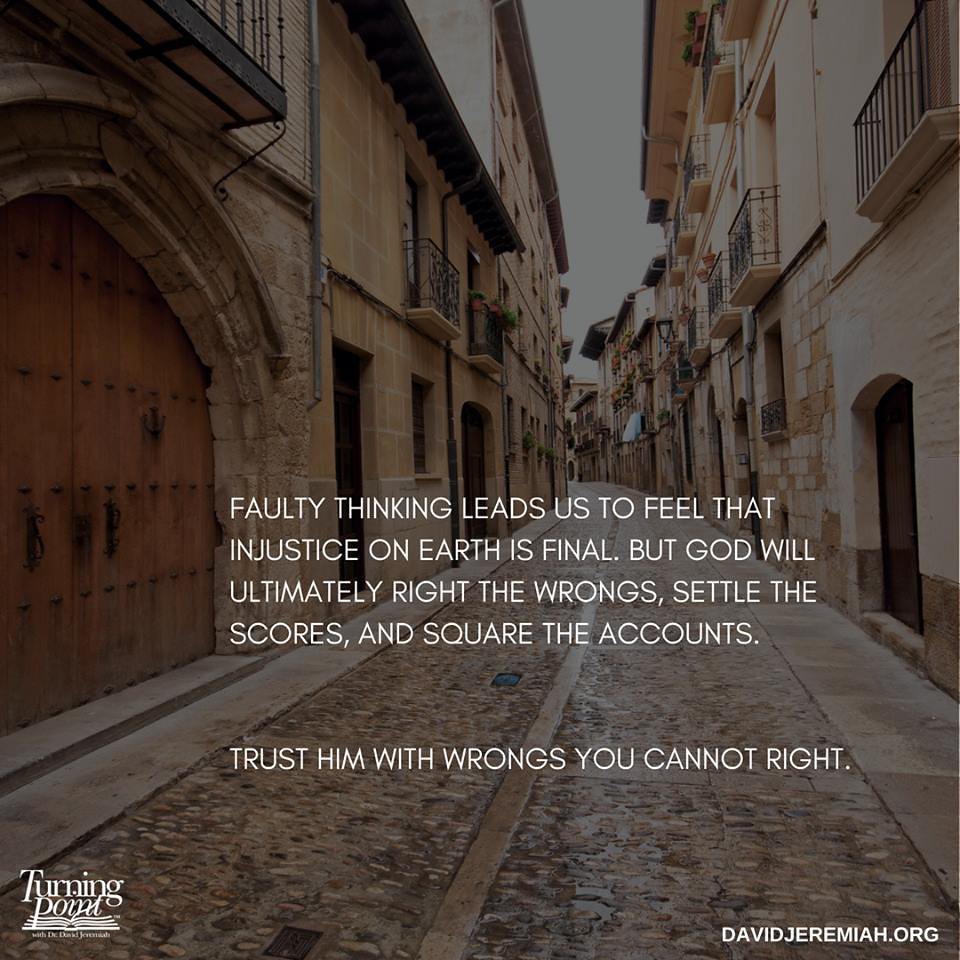The image is a religious motivational graphic depicting a dimly lit, ancient cobblestone street in what appears to be an old city, possibly Jerusalem. The street is lined with very old stone buildings, some of which have been modernized with apartments above them. The tan and cream-colored buildings feature large wooden doors and stone archways, with a particularly notable giant wooden double door with a stone archway on the left side. The cobblestones appear shiny and damp, suggesting it may have rained recently. In the center of the image, a white, uppercase caption reads: "Faulty thinking leads us to feel that injustice on earth is final. But God will ultimately right the wrongs, settle the scores, and square the accounts. Trust him with wrongs you cannot right." The lower left-hand corner displays the Turning Point Ministries logo, featuring an illustration of a book that looks like the Bible. In the lower right-hand corner, the website "davidjeremiah.org" is printed. There are no people visible in the scene.